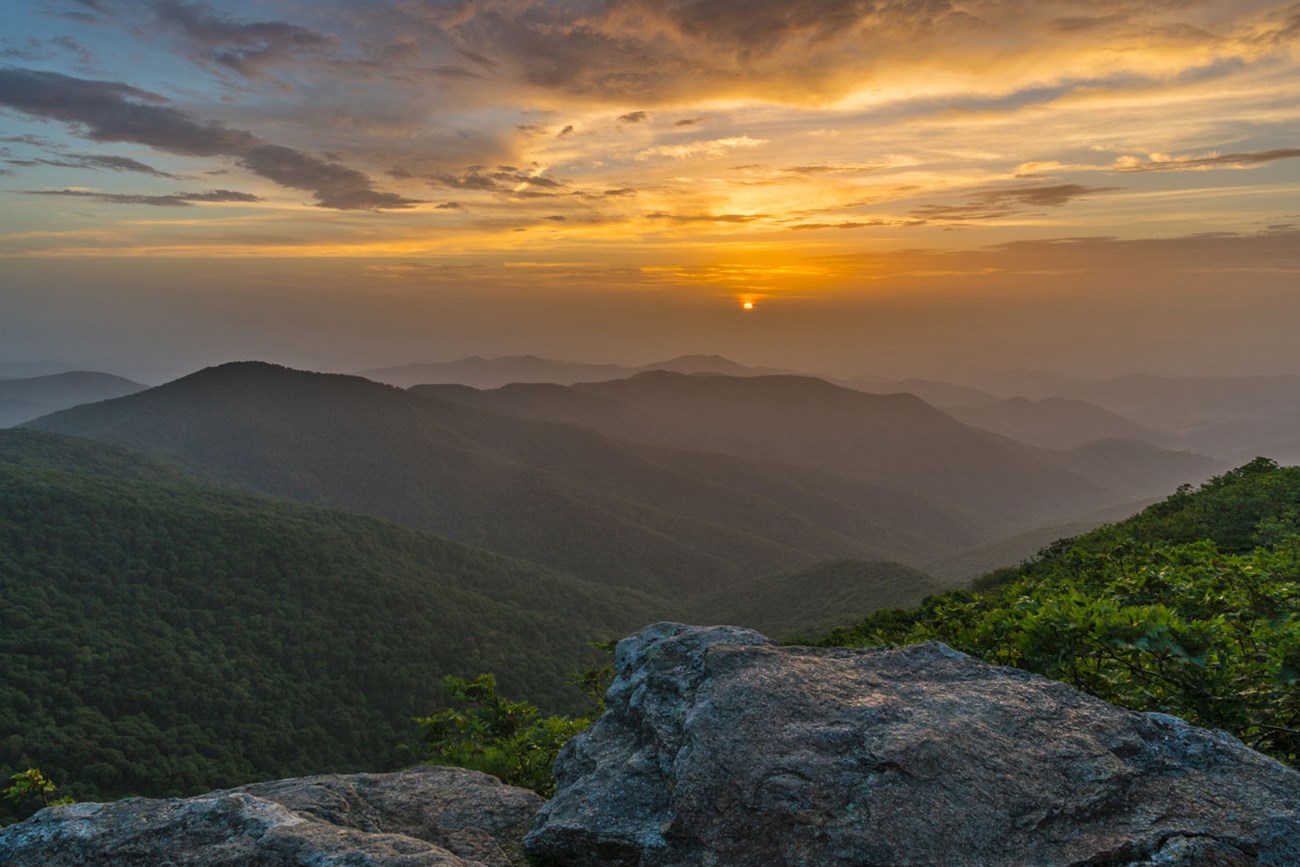The photograph showcases a stunning, expansive mountain range viewed as if from a high vantage point. In the foreground, two monumental gray granite rocks anchor the scene, suggesting the photographer is standing on one of them. Behind these rocks, lush green vegetation thrives, leading to a densely forested green hill. Further beyond, hazy, light purple hills or mountains fade into the distance, their details obscured by a mist. The sky captures the enchanting colors of a sun either setting or rising, with a small orange sun casting its warm glow. The skyline bursts with vibrant hues of orange, purple, and blue, while multiple clouds, varying from dark gray to orange due to the sun’s reflection, dot the sky. A hint of blue sky peeks through, and a subtle white halo surrounds the sun, emphasizing its brilliance in the dimming or awakening light.